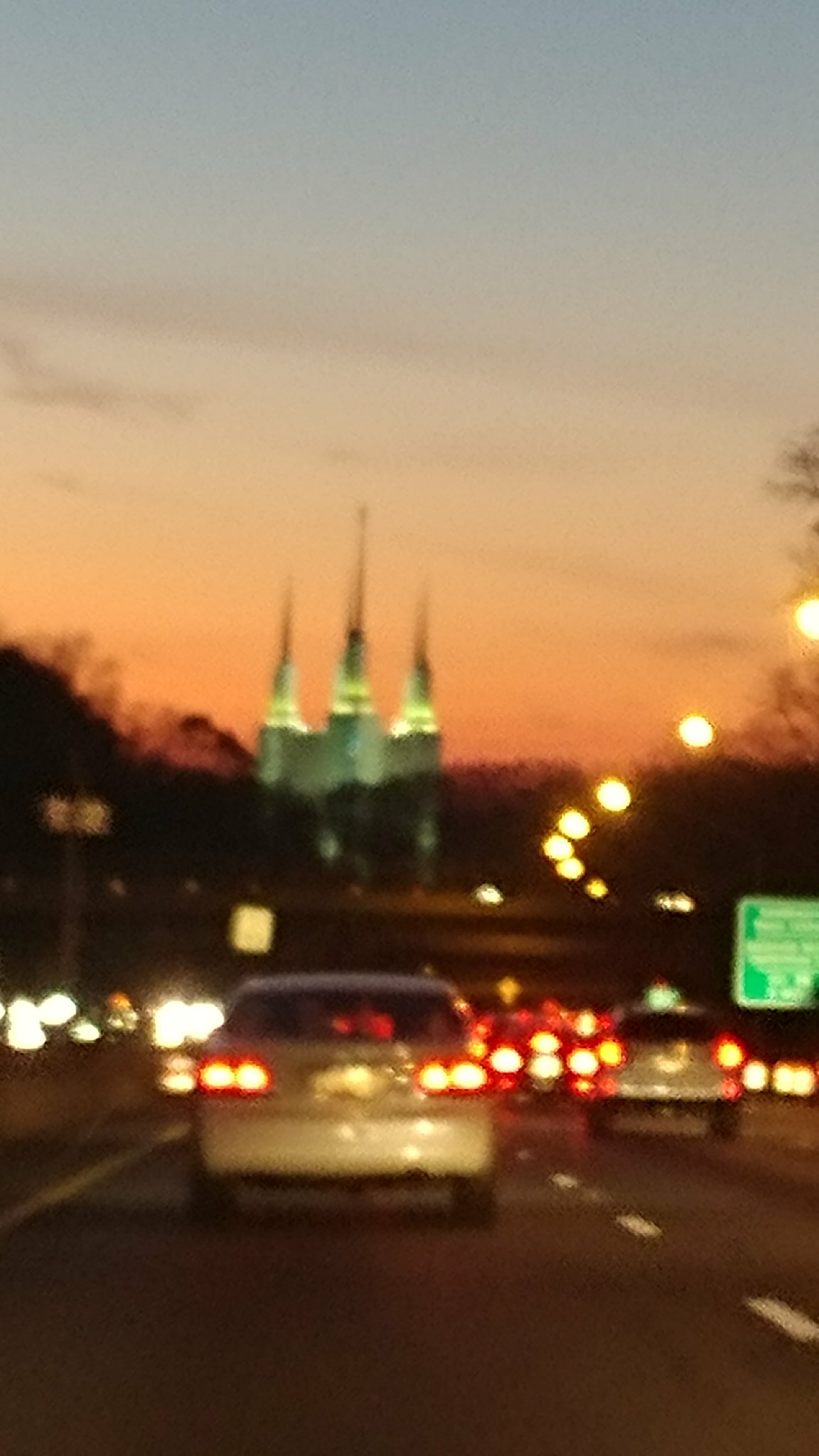At sunset, a blurred image captures a stretch of a freeway in eastern Canada. Vibrant orange hues paint the sky as dusk settles in, casting a warm glow over the scene. The taillights of cars create a trail of red light, their details indistinguishable due to the blur. On the right side, a green freeway sign stands prominently, though its lettering remains unreadable. In the distance, a stately building with steeples reaches towards the sky, likely a church or possibly a government capital building, adding a historical touch to the urban landscape.